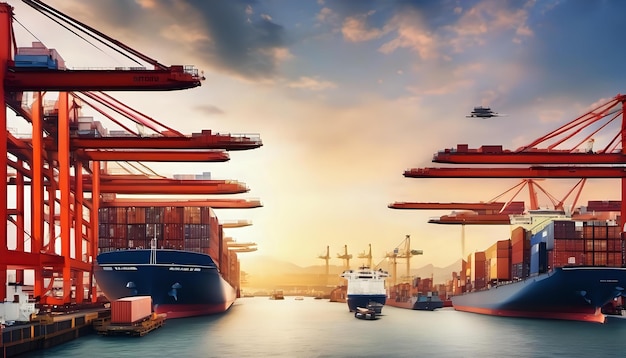The image depicts a computer-rendered scene of a bustling shipping port during sunset. Dominating the foreground are large red metal cranes on both the left and right sides, actively loading red, blue, and various colored shipping containers onto massive dark blue freighters with distinctive red hulls and white superstructures. In the center, a prominent ship with a white top and blue hull is being guided by a tugboat through a channel flanked by these cranes. The port is peppered with additional cranes and ships in the background, indicating extensive activity and scale. The ground level is a well-organized street lined with stacked containers and dotted with large forklifts and other equipment. The sky above transitions from a cloud-filled grayish-brown to a blue expanse with gray clouds, infused with an orange-peach hue, particularly on the left, where the setting sun projects a bright golden light, enhancing the scene’s vibrant, almost painting-like quality.